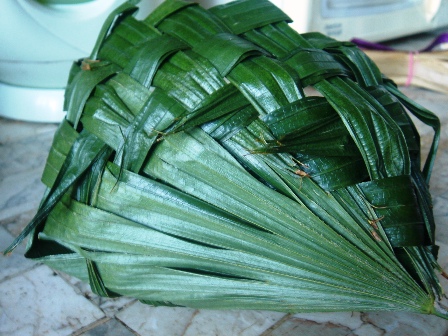The image shows a detailed, artistic arrangement of long, dark green leaves that are intricately interwoven, forming a bundle that narrows to a tip on the right. The interlacing pattern, which gives the leaves a hand-woven appearance, suggests meticulous craftsmanship. Some of the leaves exhibit lighter green shades, adding depth to the overall dark green hue. The bundle is laid horizontally from the bottom right to the upper center on what appears to be a white and gray patterned tile surface, with hints of a blue cloth in the background. The craftsmanship suggests it could be a type of vegetable or plant, possibly resembling fresh bamboo or palm leaves, though the exact type is unclear. The scene also features indistinct plastic items in the background, contributing to an intricate yet somewhat mysterious composition.